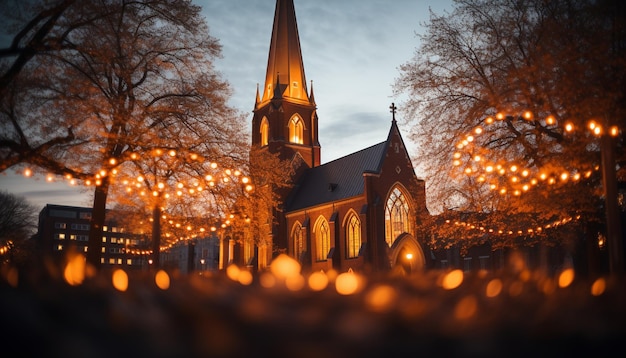This horizontal, rectangular photograph captures a beautifully illuminated church taken at dusk, just as night begins to fall. The sky is a dimming grey, providing a soft, fading light that contrasts with the vibrant illumination of the scene. The church itself stands tall and majestic, featuring a prominent steeple crowned with a cross at the center. The structure's ornate windows, which curve gracefully towards the top, glow with a warm orange light, enhancing its grandeur.

Surrounding the church are leafless trees, adorned with strings of white lights, adding to the enchanting atmosphere. These lights are most evident on the trees positioned to the left and right of the church, although similar orange lights can be seen scattered throughout the scene, including at the slightly blurred and out-of-focus foreground. To the left of the church, another building can be seen, characterized by its square, uniform windows and more straightforward architectural style, suggesting it might be separate or an annex to the church.

In the far left background, a large four to five-story building, possibly a dormitory, is visible, adding depth to the image. Overall, the church's illuminated splendor against the darkening sky, flanked by the glowing trees and additional structures, creates a striking and picturesque night-time scene.